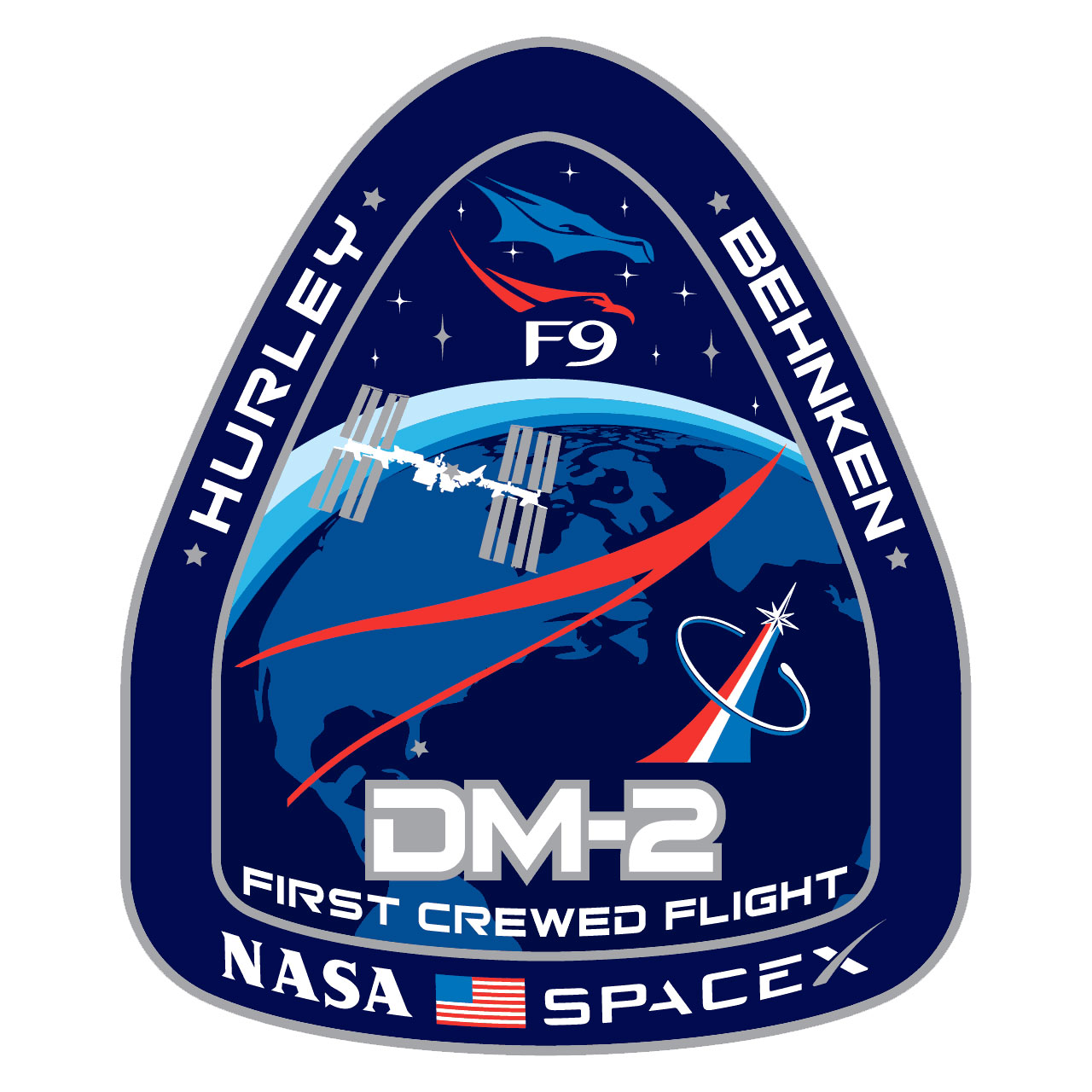This image depicts an astronaut's patch with a distinctive, rounded triangular shape that transitions into a rectangle with curved corners at the bottom. The background is dark blue, edged with a white trim that mirrors the shape of the patch. Central to the design is a detailed space scene: a white and gray outline of the International Space Station floats above a dark blue Earth, highlighted with light blue continents, showing North America clearly with a star marking Cape Canaveral.

At the top of the patch, white bold letters spell "F-9" likely referencing the Falcon 9 rocket. Prominently displayed in the center are the large letters "DM-2," with "first crewed flight" directly below it. The names "Hurley" and "Behnken" are inscribed on the left and right sides, respectively, each flanked by two small gray stars. Below, "NASA" and "SpaceX" are printed, separated by a small American flag.

Overall, the patch serves as a detailed and symbolic representation of a milestone space mission, blending astronaut names, mission identifiers, and national pride into its complex design.